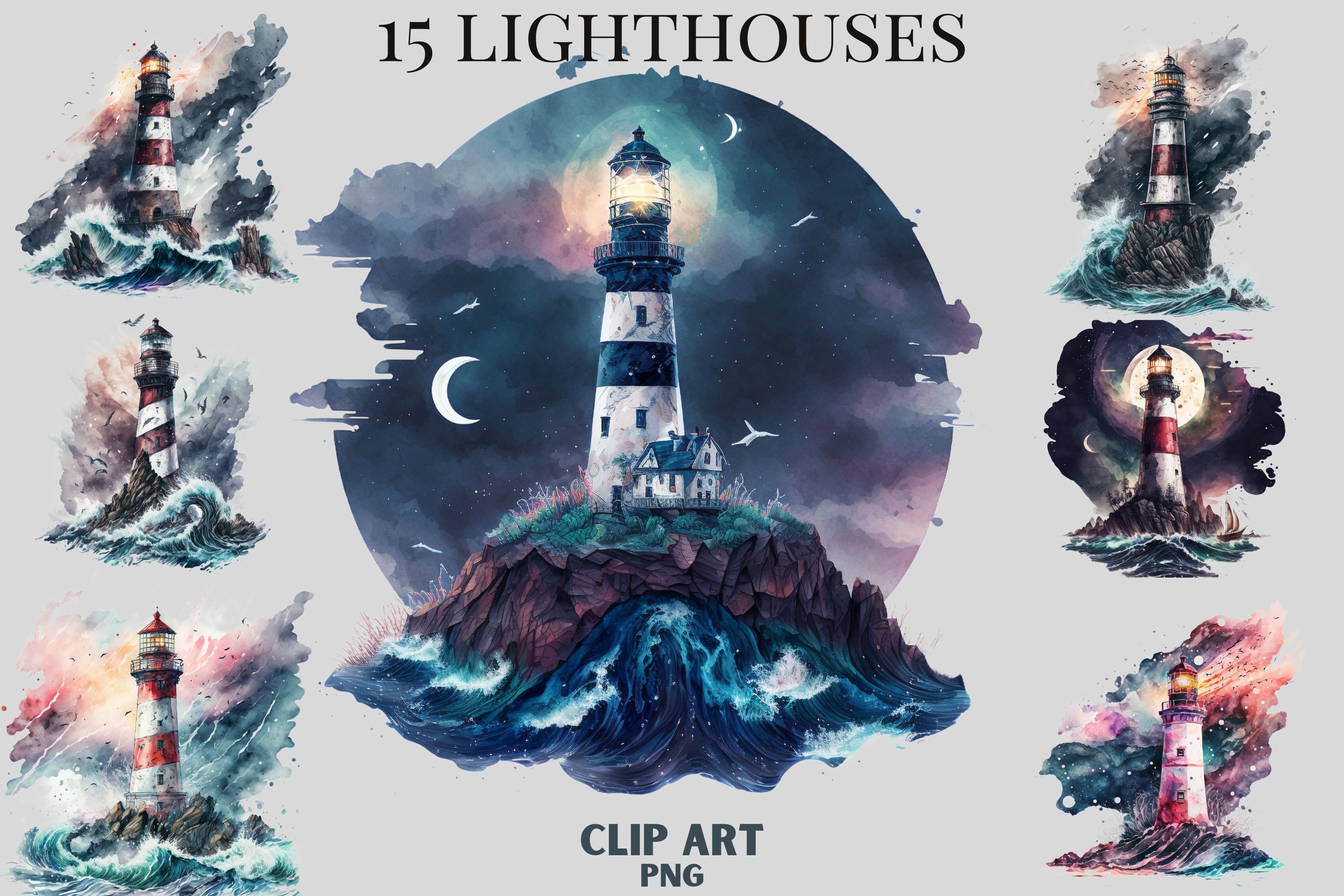This detailed digital artwork resembles the front cover of an art book or a poster, titled "15 Lighthouses" at the very top in black letters. At the bottom, it reads "Clipart PNG" in silver. The central focus is a large lighthouse depicted in blue with white stripes, standing on a small rocky island amidst stormy waters, and backed by a bright, full moon in a nighttime setting.

Flanking this prominent lighthouse, on both the left and right vertical edges, are smaller lighthouses—each uniquely designed and placed within its own vignette against an off-white, almost gray background. The left side features three smaller lighthouses: the top one with horizontal red and white stripes, and the other two with diagonal red and white stripes. The right side mirrors this arrangement but includes variations: the top right lighthouse shares the horizontal stripe design, the middle one is predominantly white with a singular large red stripe near the top, and the bottom right lighthouse is colored in pink.

Each of these smaller lighthouses appears to be set against abstract, undefined backgrounds, with watery and rocky elements suggesting wave action, enhancing the isolated, picturesque aura of the scenes. These backgrounds do not have the cohesive cloud globe effect that surrounds the central lighthouse.